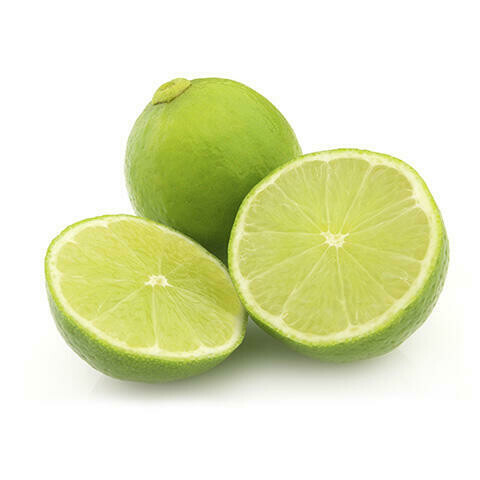This image features three pieces of ripe lime set against a plain white background, creating a sharp contrast that highlights the vibrant colors of the fruit. At the center back of the image, there is a whole, intact lime with bright neon green skin, indicating its ripeness. In the foreground, a lime has been sliced in half, revealing the light minty green flesh inside. The cut lime halves are placed side by side, showcasing the detailed inner structure with multiple triangular segments radiating towards a central white dot. The outer peel of these halves matches the bright green of the whole lime. The overall composition, with its simple and clean background, makes this a vivid and colorful image that could serve effectively as a product photo for an online grocery store. The drop shadow at the base adds a subtle depth to the otherwise flat scene, enhancing the fresh and appealing presentation of the limes.